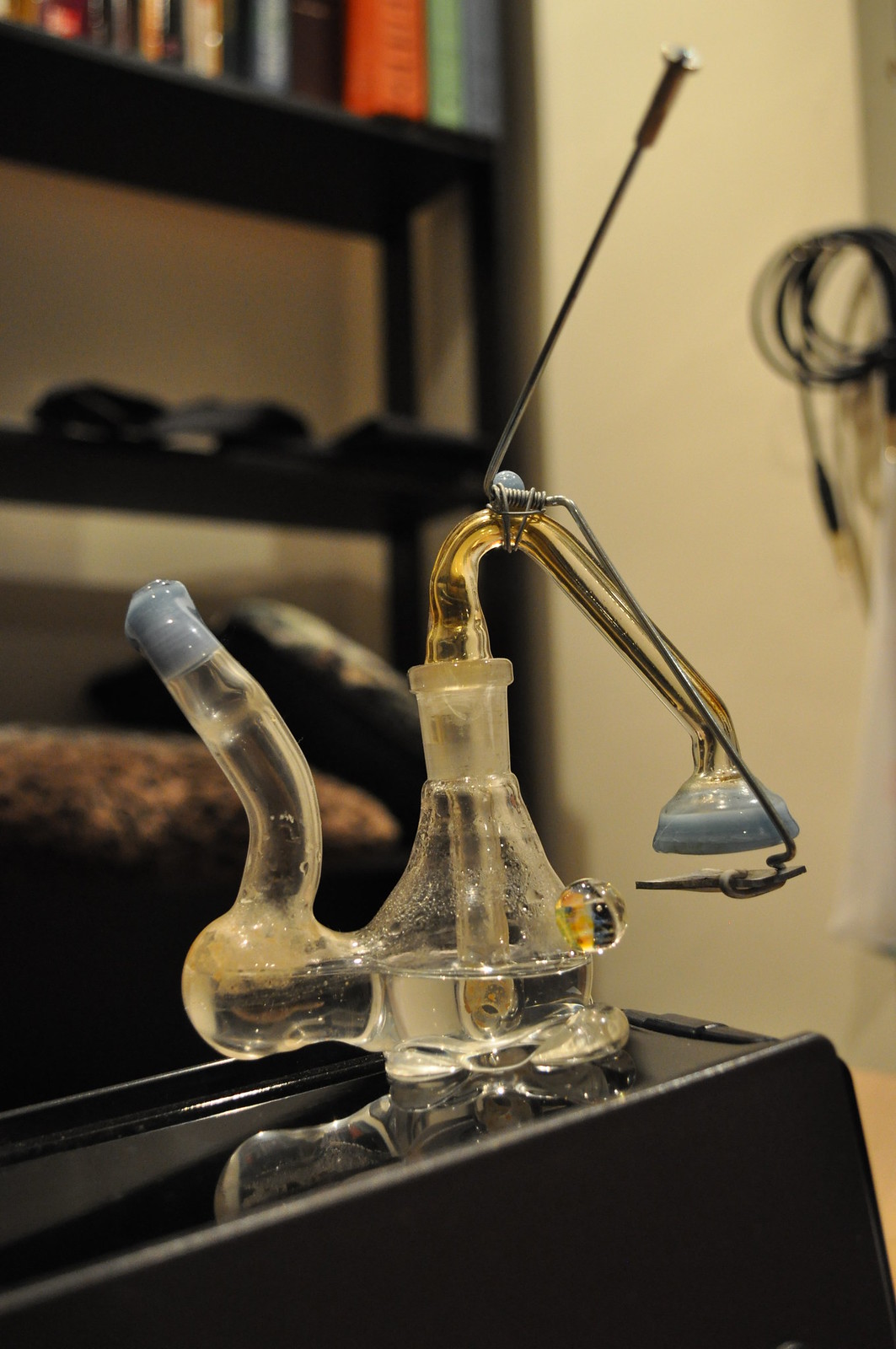In the center of the image is a complex glass apparatus, likely a dab rig or some sort of scientific device, comprised of multiple connected glass vials and tubes. The main component appears to be a glass flask partially filled with water, featuring a tube that extends inward. A curved tube emerges from this flask and loops downward. This structure rests on a shiny black surface with raised borders on its left and right sides. The setting seems to be a cluttered indoor space, possibly a bedroom. The background is blurry but discernible, featuring a black bookshelf filled with a colorful assortment of books arranged as follows: red, blue, green, red, black, blue, black, pale brown, black, pale brown, black, black, red, and yellow. Additionally, black wires are seen coiled and hanging in the upper right corner of the image. Overall, the image contains no text and showcases a mix of colors, including tan, red, green, black, maroon, orange, gray, light blue, silver, and pale brown.